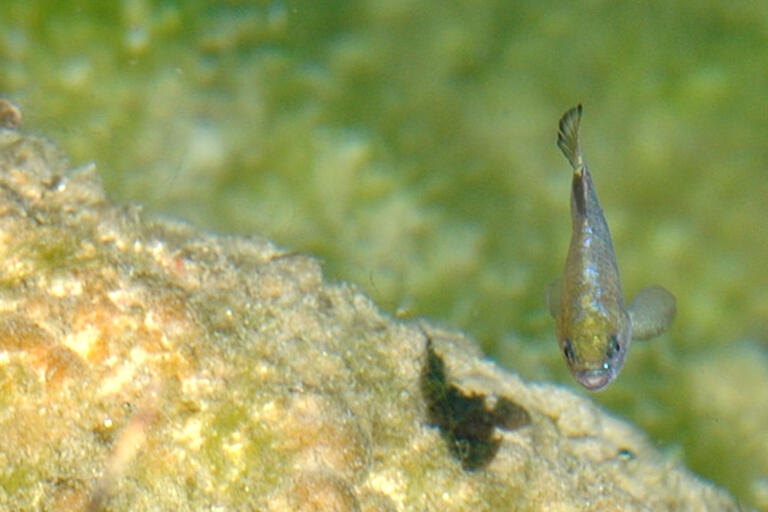This underwater photograph captures a small fish swimming in a blurred, tranquil aquatic environment. The image is taken from above, showing the fish moving forward and casting a distinctive black shadow to its left. The fish is primarily silver with a notable greenish-yellow spot on its head and a tail fin that transitions to black. The foreground features a small, textured hill composed of greens, browns, and subtle hints of sediment, suggesting the presence of fish eggs or rocks. The hill adds depth to the scene, while the background remains a soft blur of green, blue, and white hues, emphasizing the serene underwater setting.